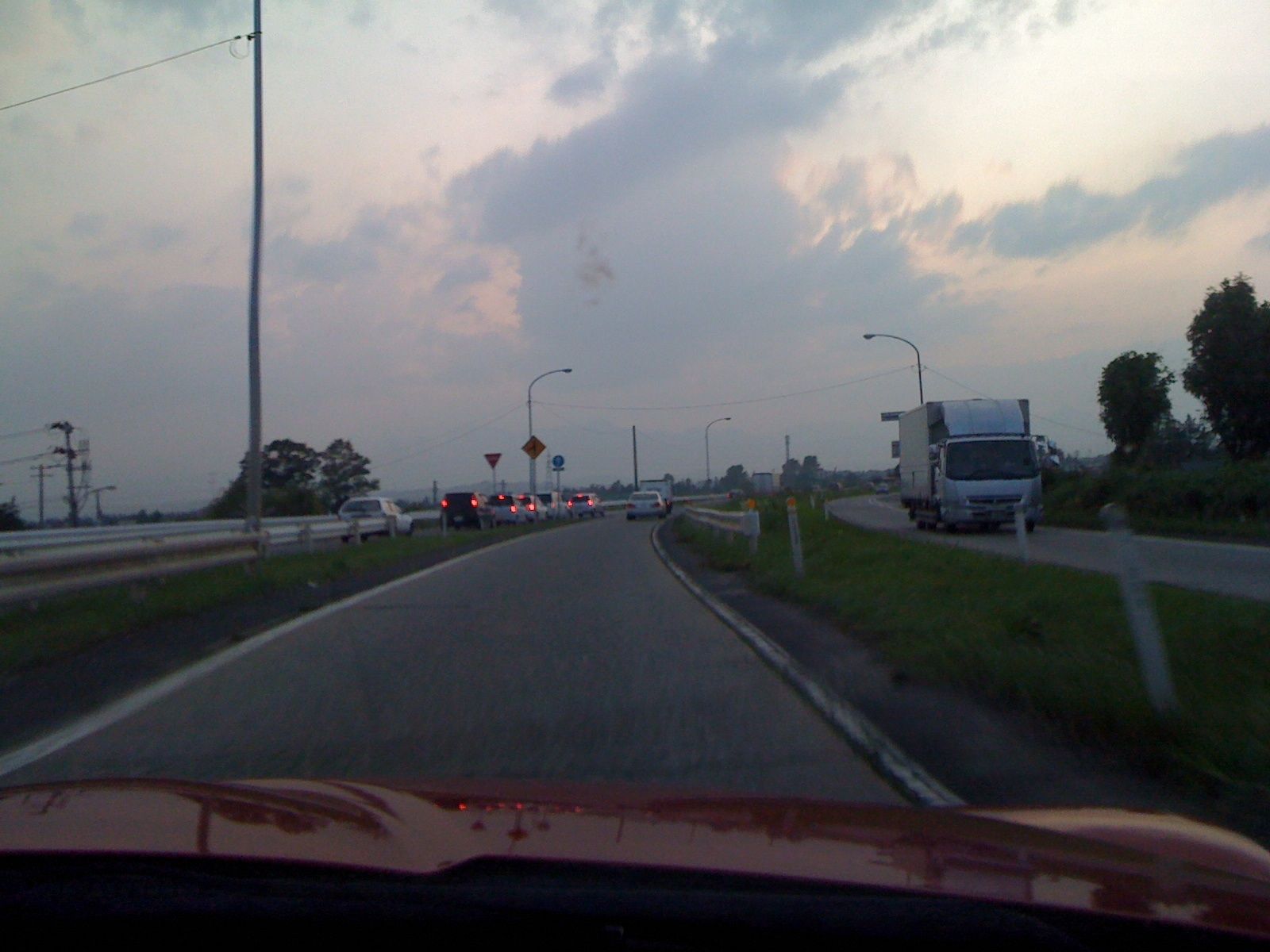The image inside the car showcases a detailed view over the black dashboard and the red hood, indicating the vehicle's presence on a road. The windshield reveals a multi-lane highway scene with three lanes: one merging lane, one main traffic lane heading in the same direction, and a lane for oncoming traffic. The sky, a rich blue interspersed with splayed clouds and hints of sunlight, looms over a landscape dotted with light poles and various trees. A small truck is visible on a separate, grassy-divided road heading toward the viewer. The road has accompanying street signs and patches of grass both alongside it and in the median, which also features light poles and a guardrail. Several cars travel in the same direction on the main highway, and some appear to have their lights on, likely indicating dusk with the street lights yet to be activated. The reflections off the car’s red hood capture elements of the sky, clouds, and nearby traffic, further enriching the twilight scenery.